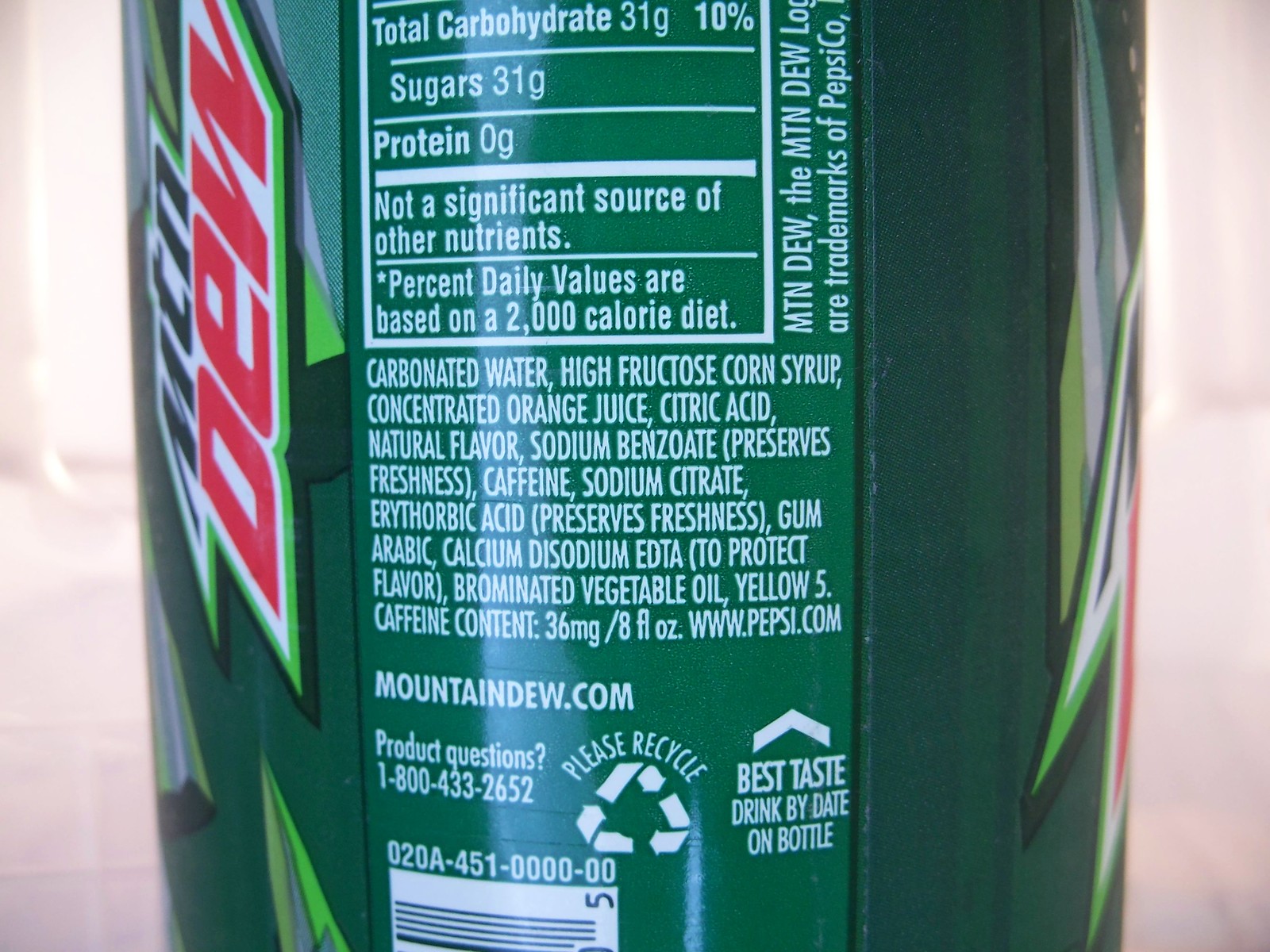This image portrays the side view of a bottle or can of Mountain Dew, highlighting various details primarily from the nutritional information and packaging labels. The label begins with the nutritional facts: Total Carbohydrates at 31 grams, accounting for 10% of the daily value, and Sugars also at 31 grams. The Protein content is listed as 0 grams, and it notes that this beverage is not a significant source of other nutrients. The Percent Daily Values are based on a 2,000 calorie diet.

The ingredients start with carbonated water and high fructose corn syrup, among other listed components. The bottom section of the label provides additional information, including the official website (mountaindew.com) and a customer service phone number. It also encourages recycling and mentions a best taste date, though the date itself is not visible in this image.

The packaging is visually striking with a green background and red lettering for the "Dew" logo, adding to its iconic branding.